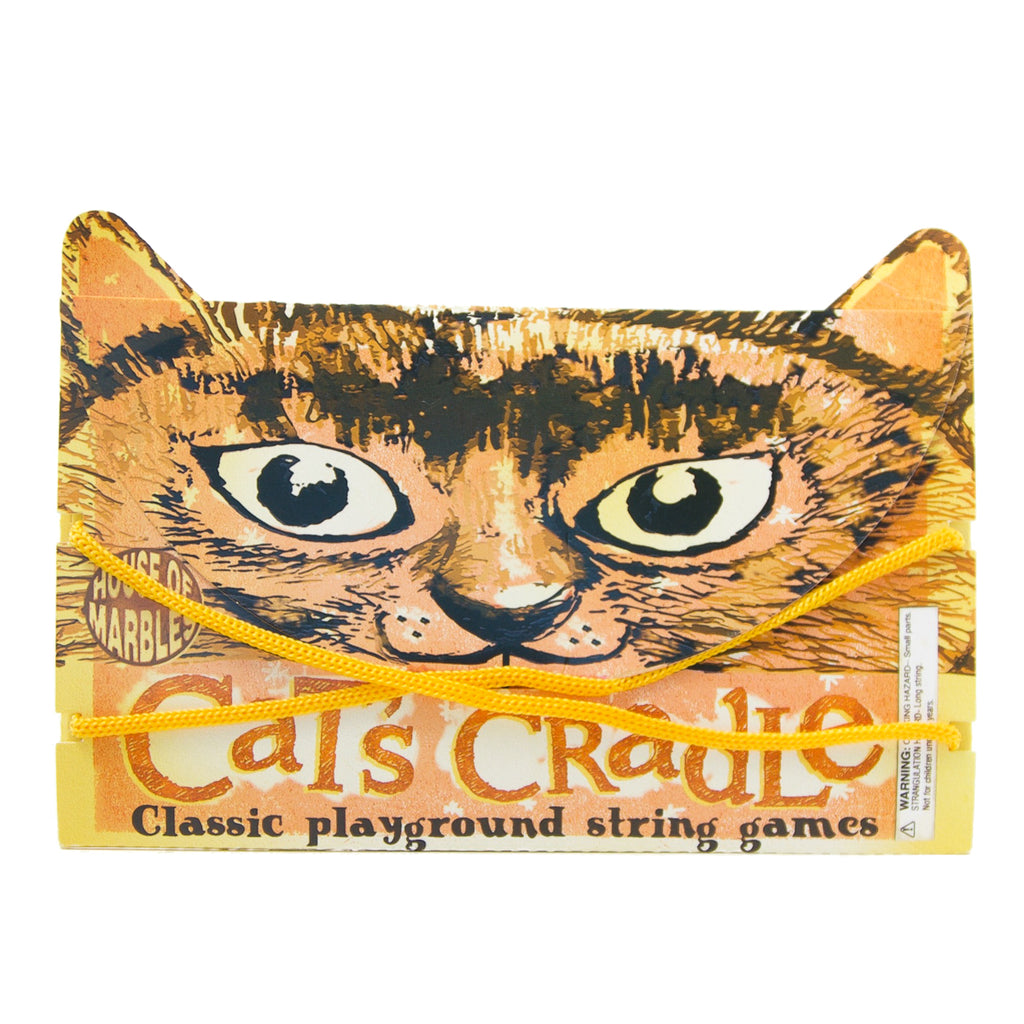The image depicts a retro-styled packaging for the classic children's toy, Cat's Cradle. The rectangular package features a predominantly yellow and orange cartoon-like depiction of a cat's face, complete with white eyes and black pupils, and its black ears extending into a white background at the top left and right corners. Two yellow strings cross diagonally across the front, from the middle left to bottom right and from the middle right to bottom left. On the left side of the packaging, there is a circular brown logo with yellow letters that reads "House of Marbles." At the bottom of the package, "Cat's Cradle" is prominently displayed in orange lettering on a white background, with "Classic Playground String Games" written below in black. The packaging also includes a warning hazard label, indicative of its child-oriented design. The overall aesthetic of the product gives off a nostalgic, retro vibe, reminiscent of designs from the 1960s.